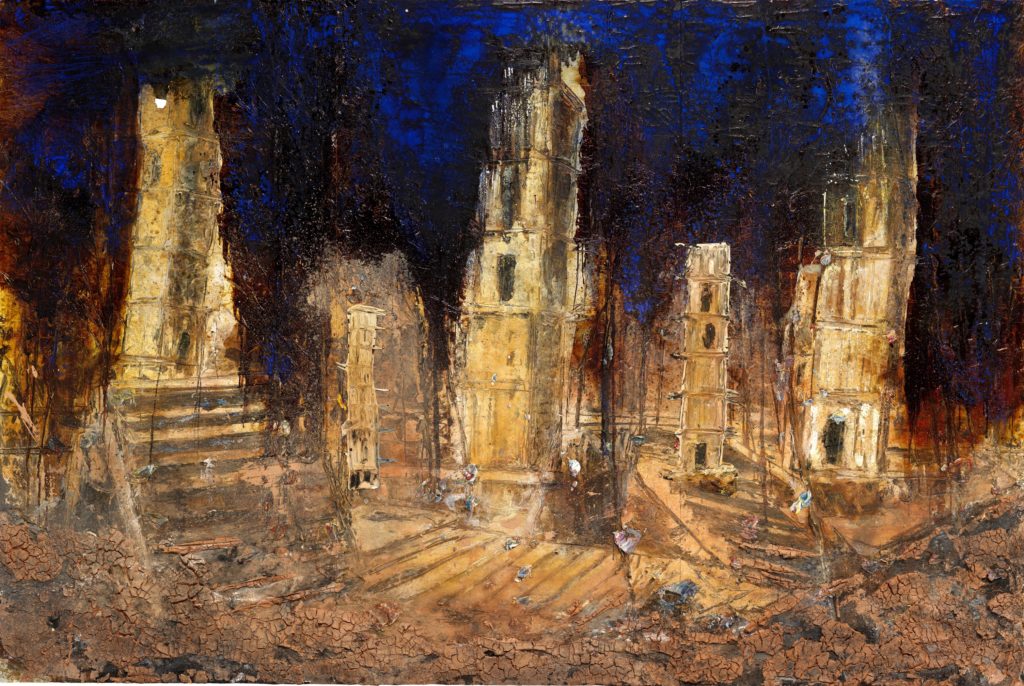The painting portrays an impressionistic cityscape dominated by a foreboding dark black and blue sky, creating an illusion of night. The composition centers around a series of buildings and towers that appear to be in various stages of ruin, reminiscent of bombed-out relics from a past era, akin to structures subjected to wartime destruction. In the foreground, features such as streets and staircases blend into the scene, rendered in earthy tones like brown, light brown, and green. These colors form a stark contrast with the dark sky above. The tactile texture of the painting is enhanced by cracked paint at the bottom, deliberately suggesting debris and ruin. The overall effect is a shimmering, almost glowing portrayal of industrial blight—an apocalyptic vision that combines both chaos and melancholic beauty.